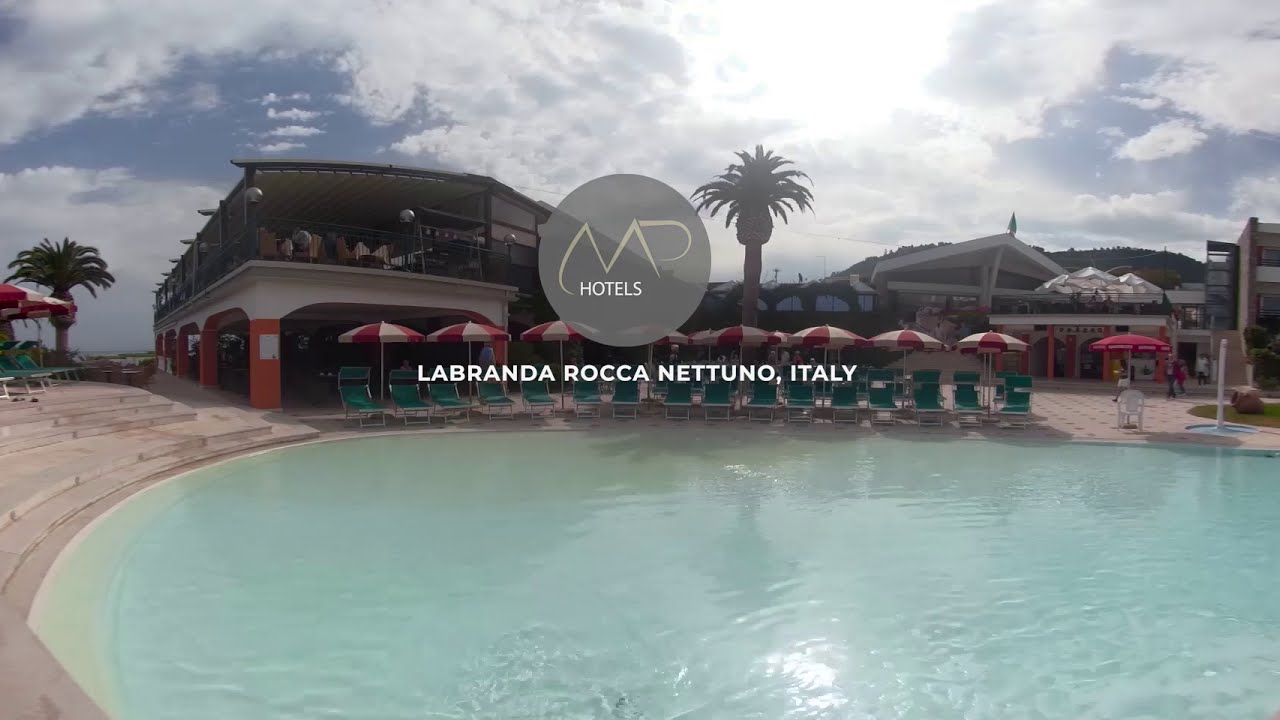This photograph showcases an inviting scene of an oval-shaped, crystal-clear blue pool, likely at a resort or public facility. The turquoise-hued water gently ripples under a dull blue sky filled with scattered white clouds, punctuated by a bright orb of sunlight. Surrounding the pool, you’ll find concrete steps leading into the water, lined with teal-colored chairs and red-and-white umbrellas, though none are occupied. The setting appears serene and quiet, with a few individuals emerging from a two-story building situated directly adjacent to the pool. The building features distinctive white and red arches and includes a balcony on its upper level, presumably housing restaurants. Towering palm trees add a touch of exotic greenery to the scene. Dominating the center of the image is a transparent gray circle displaying the light yellow and white MP Hotels logo, accompanied by the text “LABRANDO ROCCA, NETUNO, Italy” in capital letters below.